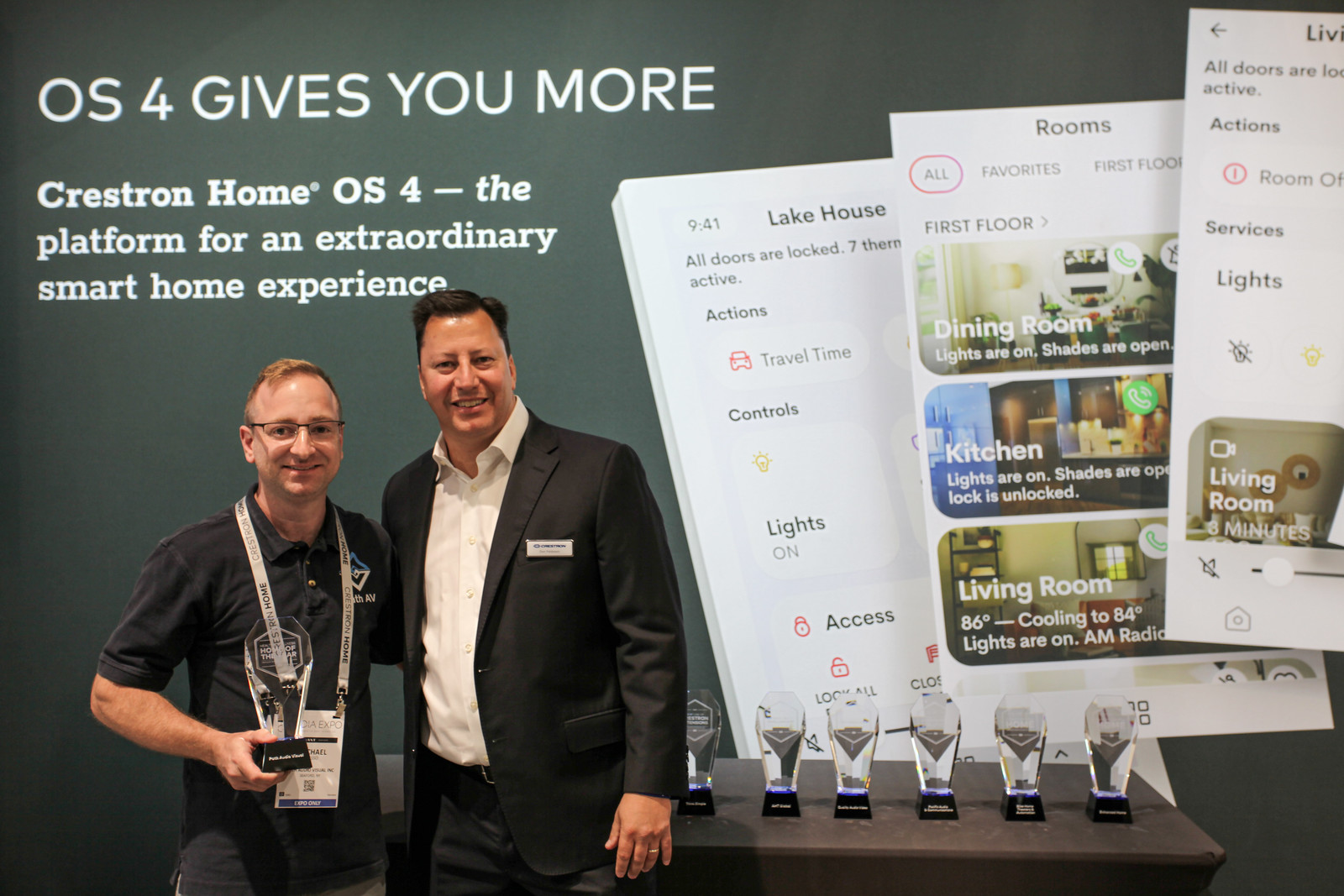In this rectangular, horizontally oriented image, set against a darker gray background, we see two men standing in front of a table displaying multiple glass awards with black bases. The awards appear to be accolades for smart home technology, possibly labeled "Honor of the Year" or "Home of the Year." 

In the upper left-hand corner, white text prominently reads: "OS4 gives you more, Crestron Home OS4, the platform for an extraordinary smart home experience." The man on the left, identified by his white name tag as Michael, is holding one of the glass awards in his right hand. He is a slender figure, wearing a black short sleeve shirt and dark gray jeans, and he has glasses and a noticeably large nose. He smiles at the camera.

To Michael's right stands a larger man dressed in a black sports coat and white button-up shirt with dark pants. He has his arm around Michael, and both men are smiling warmly at the camera. 

To the right of the men, atop a short brown table, lies a collection of similar glass awards. Additionally, in the upper right corner of the image, there are pamphlets showcasing various home scenarios like the dining room, kitchen, and living room, which likely describe the smart home capabilities facilitated by Crestron Home OS4.